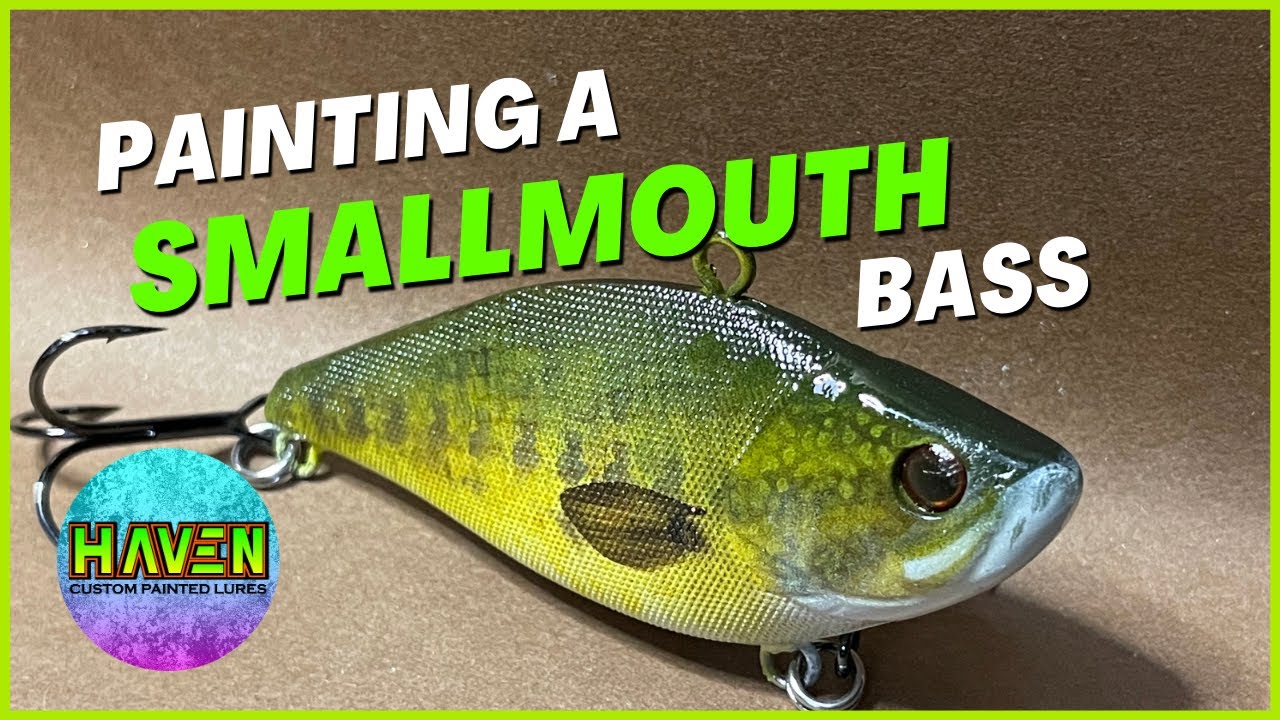This image is a staged, promotional, full-color photograph with digital enhancements, depicting a custom-painted fish lure designed to resemble a smallmouth bass. The horizontally rectangular image is bordered by a thin lime green line and is set against a brownish-beige background, adding a photographic realism combined with graphic design typography. The fish lure is centrally positioned near the bottom half of the image, orientated with its face pointing to the bottom right and its tail to the bottom center-left. The lure features dark green scales with speckles, a yellow underbelly, and brown eyes, complete with multiple hooks: one on its back, a couple near its mouth, and a three-pronged hook at the tail. 

Above the lure, the text reads "painting a" in white, followed by "small mouth" in bright green, and "bass" in white, all arranged on a slight angle. In the lower left-hand corner, there is a circular logo that gradients from light aqua at the top to purple at the bottom, containing the word "Haven" in bright green text, outlined in red, and beneath that, "custom painted lures" in black text. This detailed composition effectively highlights the fish lure, making it visually appealing for promotional purposes.